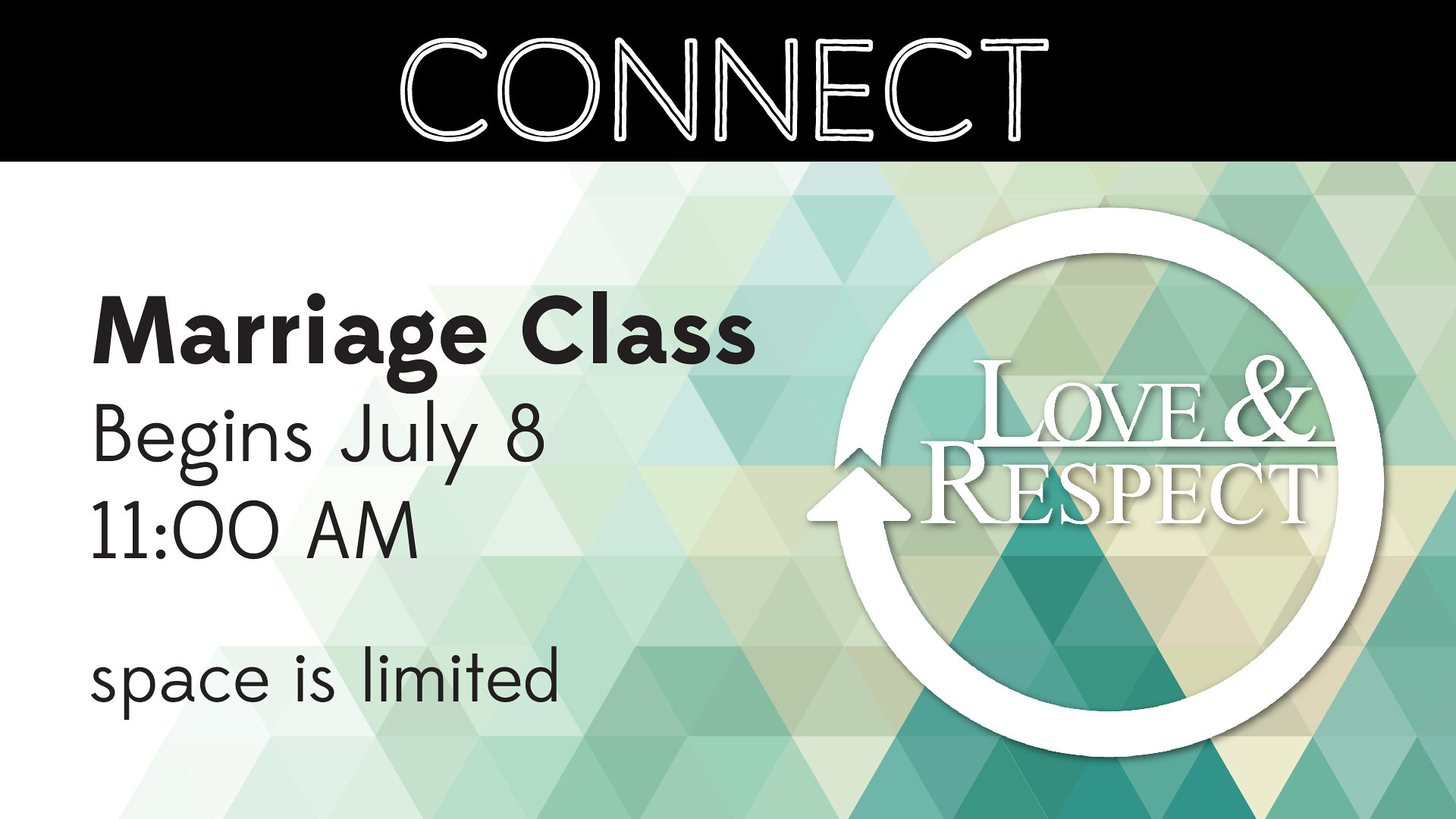The image is an advertisement with a distinct black band running along the top, featuring the word "CONNECT" in bold, centered white letters. Below this, the background transitions from a light color on the left to a green ombre on the right. The left side of the image features a series of intersecting triangles in varying shades of grey and yellow, enhancing the design's complexity. In bold black text on the left, it declares, "MARRIAGE CLASS BEGINS JULY 8 11 A.M. SPACE IS LIMITED." On the right side, there's a white ring formed by an arrow that loops back on itself. Inside this ring, in bold white capital letters, it reads "LOVE & RESPECT." The entire background begins as white on the far left, gradually shifting to a more pronounced green as it moves to the right.